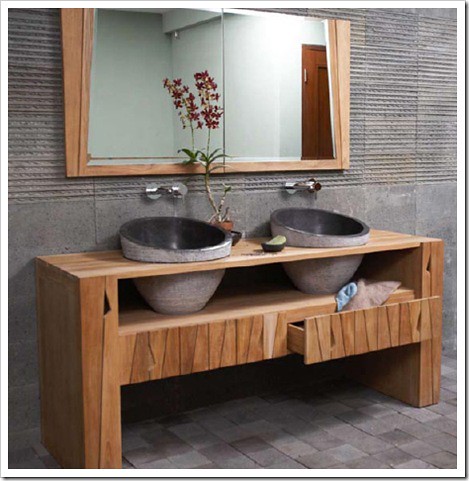The image captures a modern bathroom with a striking gray wall serving as the backdrop. Intricately designed, the bathroom features multiple built-in niches. At the center is a large mirror framed by a white wall and a brown door located to the right.

Flanking the left and right sides of the sink area are stone bowl sinks positioned atop a counter. Each sink is paired with a sleek, silver faucet, depicted in mid-motion, pouring water into the stone bowls beneath. 

Central to the vanity is a decorative vase containing various stems, surrounded by lush green foliage that adds a natural touch to the space. At the top of the foliage, vibrant red flowers provide a pop of color amid the greenery.

Elements of wood are interspersed throughout, including thick wooden panels on both the left and right sides of the bathroom. An open drawer on the right-hand side hosts some neatly folded blankets spilling out.

The floor is a blend of gray and blue tiles, with a mix of light gray, dark gray, and very dark tiles creating an intricate pattern. Across the top of the image, multiple lines traverse, adding to the architectural interest of the room.